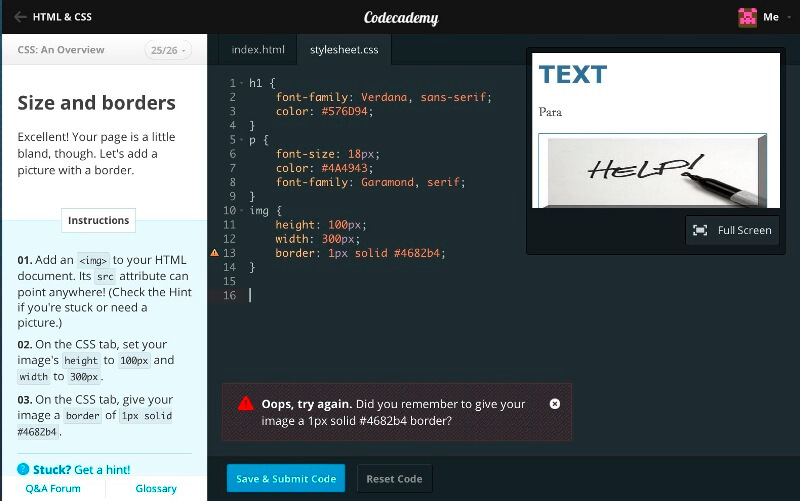The web page from Code Academy prominently features a top banner with "Code Academy" written in an elegant semi-cursive white font. On the left sidebar, there are selectable options for HTML and CSS courses. The current section is titled "CSS Overview," specifically focusing on "Size and Borders," as indicated by the progress (25 of 26 lessons completed). The interface includes a motivational message, "Excellent. Your page is a little bland though. Let's add a picture with a border," followed by step-by-step coding instructions.

A feature allowing users to request help, such as “Stuck? Get a hint,” is available, along with additional support options like a Q&A forum and a glossary. Underneath the "Code Academy" banner, there's a code editor section where users input their code. Adjacent to this, a preview panel shows the resultant image with text, complemented by a clickable “help” button for further assistance.

The overall color scheme of the web page is a sleek black background, with the instructional text highlighted in a light blue background for better visibility. An error message reads, "Oops, try again. Did you remember to give your image a one-pixel solid border?" prompting the learner to correct their code accordingly. The instructional area uses a contrasting white background with black text for clarity.